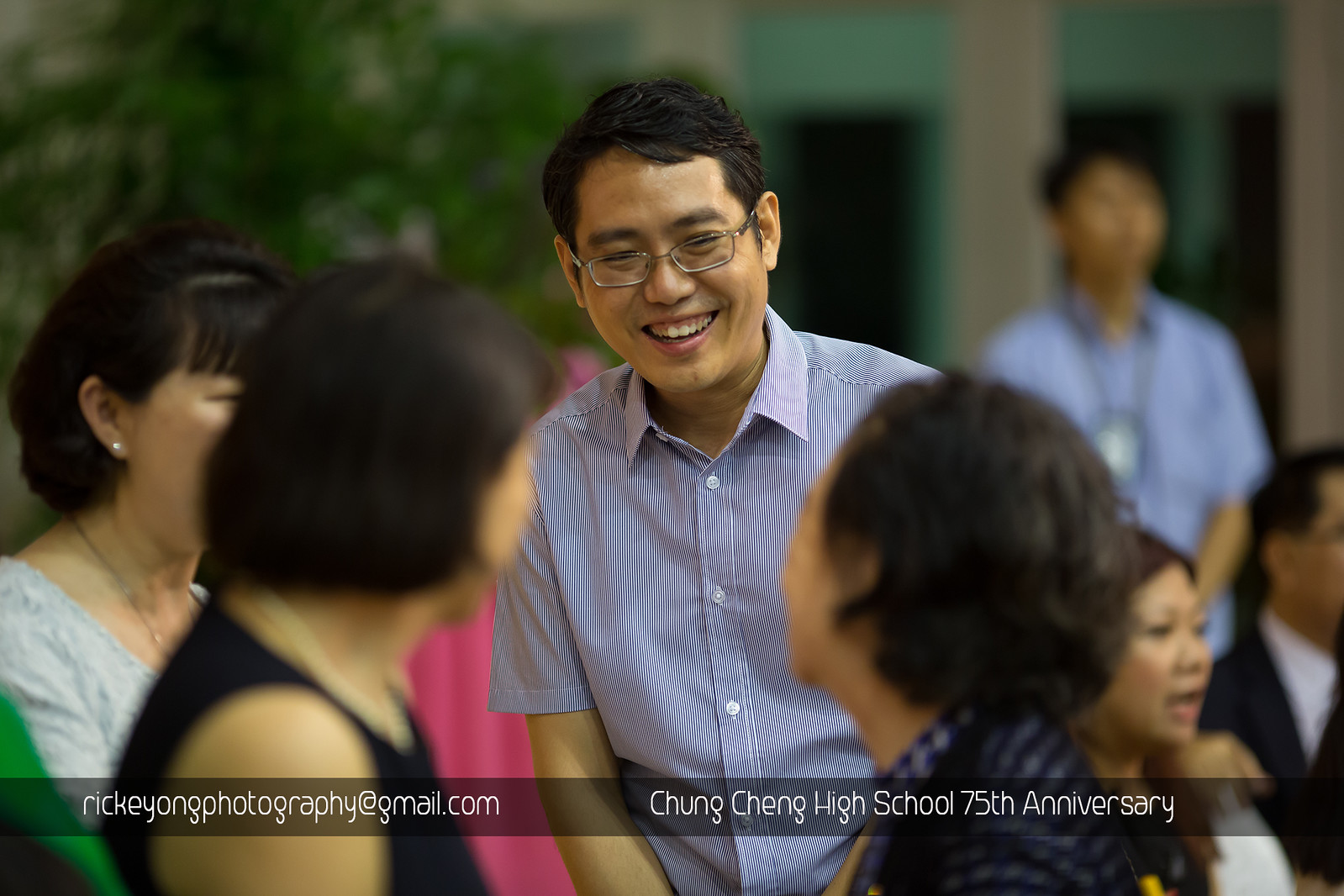This photograph captures a vibrant scene featuring a group of Asian individuals, prominently centered around an Asian man with short hair and glasses, smiling warmly. He appears to be in his 30s or 40s and is dressed in a blue and white striped, short-sleeved button-up shirt. 

In the foreground, two women with medium-length hair can be seen from behind; the woman on the left is wearing a black top, while the woman on the right is in a long-sleeved shirt. Both women's heads appear slightly blurry due to the camera's focus. To the left of the smiling man, another woman with medium-styled hair is visible, dressed in a white dress. 

On the right side of the image, a blurred, short-sleeved Asian man partially appears, enhancing the depth of the scene. In the background, the room is slightly out of focus, but a young man in a blue shirt can be distinguished, adding to the ambiance of the gathering.

Overlaying the image at the bottom is some Asian text and an email address ending with gmail.com. The bottom right corner features the text "Chong Cheng High School 75th Anniversary," emphasizing the celebratory nature of the event.